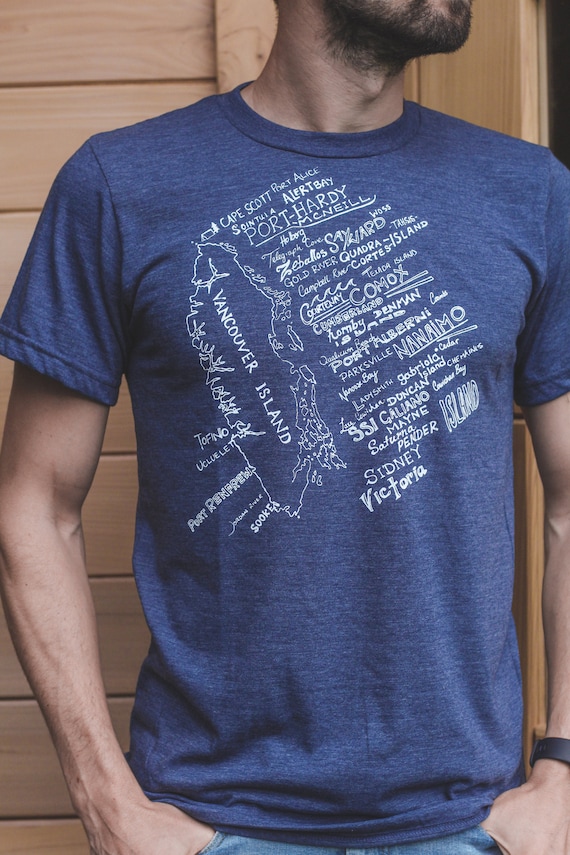The image is a portrait-mode photograph of a light-skinned man standing on top of a wooden building, modeling a blue t-shirt with a black beard and his face turned towards the right, making his facial features indistinguishable. He is wearing a light blue t-shirt adorned with a detailed map of Vancouver Island. On the left side of the shirt, several towns such as Tofino, Ucluelet, Port Renfrew, and Jordan River are listed in white letters, while on the right side, the t-shirt features more names like Cape Scott, Port Alice, Sointula, Alert Bay, Port Hardy, and Port McNeill. The names are displayed in both script and normal font, accompanied by small illustrations of a tent and tree. The man has his hands in his jean pockets, with a black watch visible on his left wrist. The image is of a real man from the neck down, emphasizing the t-shirt and its design.